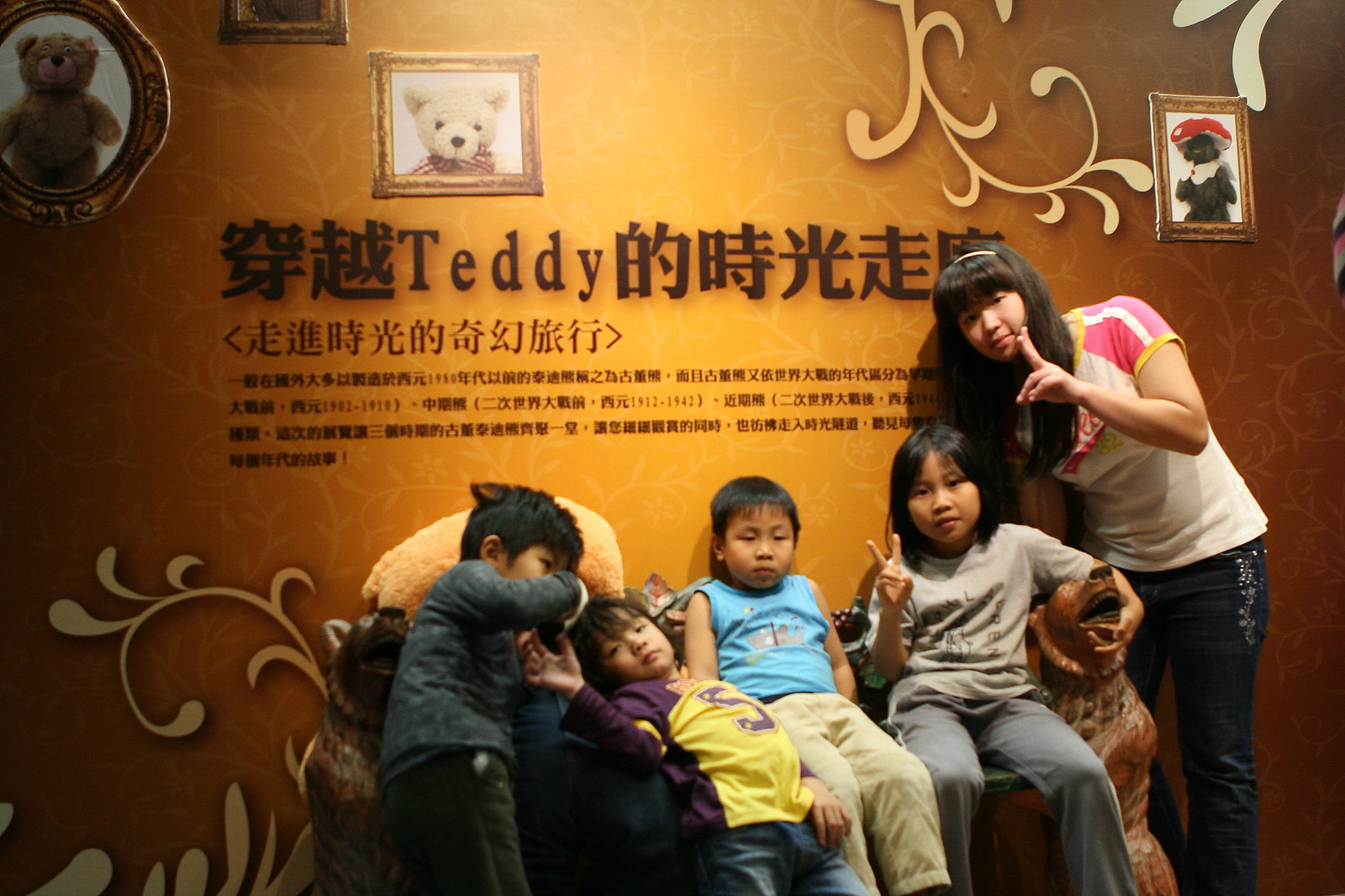In the photograph, an Asian woman with long black hair, wearing blue jeans and a white top with pink short sleeves, adorned with a white headband, stands next to four Asian children. Two of the children and the woman are making peace signs. The children, dressed in various colors, are relaxedly draped across a stylized curved bench supported by carved wooden statues of wolves. Positioned alongside the woman, the children include a girl in a purple and yellow jersey, a boy in a sleeveless blue top, another boy in khaki pants, and a girl wearing a beige t-shirt with grey pants. In the backdrop, a yellow wall is adorned with the word "teddy" in English, surrounded by Chinese characters and images of teddy bears, one notably wearing a mushroom hat. The display includes dates ranging from 1912 to 1962, possibly indicating ancestral memorials. The lighting highlights the five central figures against the intricate details of the bench and the decorative wall.